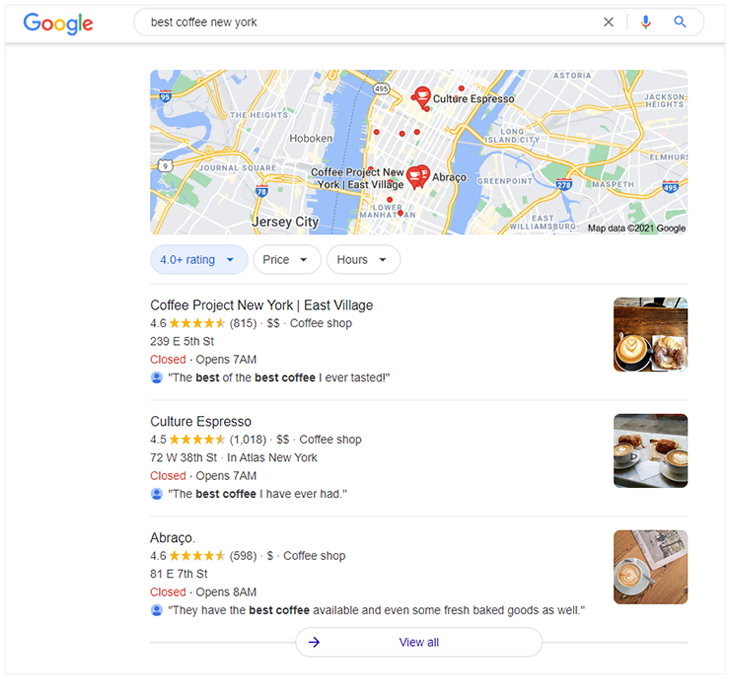Screenshot of a Google search for "Best Coffee, New York":

This large, square image features a clean, white background. At the top left corner is the iconic Google logo. Adjacent to the right sits the search bar, populated with the text “best coffee, new york” in lowercase block letters. To the right of the search bar are the familiar icons: an 'X' to clear the search, a microphone symbol for voice search, and the magnifying glass search button.

Directly below the search bar, occupying a vast area at the top of the results, is a large rectangular map of New York City. Scattered across the map are red icons emblazoned with coffee cups, indicating the location of top-rated coffee shops.

Beneath the map, to the left, are three clickable filter options: “Rating” (defaulting to 4.0 and above, with a dropdown), “Price” (with two dollar signs indicating moderate pricing), and “Hours” (with another dropdown).

Here’s a detailed breakdown of the top three listings as they appear on the left under the map:

1. **Coffee Project, New York, East Village**:
   - **Rating**: 4.6 stars out of 5 from 815 reviews.
   - **Price**: Two dollar signs ($$).
   - **Category**: Coffee Shop.
   - **Address**: Listed under the name.
   - **Hours**: Displayed with open/close times.
   - **Review**: A brief, user-submitted review.
   - On the right: A user-uploaded photo associated with the listing.

2. **Culture Espresso**: Follows the same format as the Coffee Project listing, providing a snapshot of ratings, price, category, address, hours, and a user-submitted review accompanied by a user photo.

3. **Abricot**: Similarly structured, this listing includes all key details such as ratings, price, category, address, hours, and a user review, paired with a representative user-uploaded image.

This detailed and organized layout ensures that users can easily compare top coffee spots in New York, guided by ratings, pricing, and user reviews, while providing visual insights through posted photos.